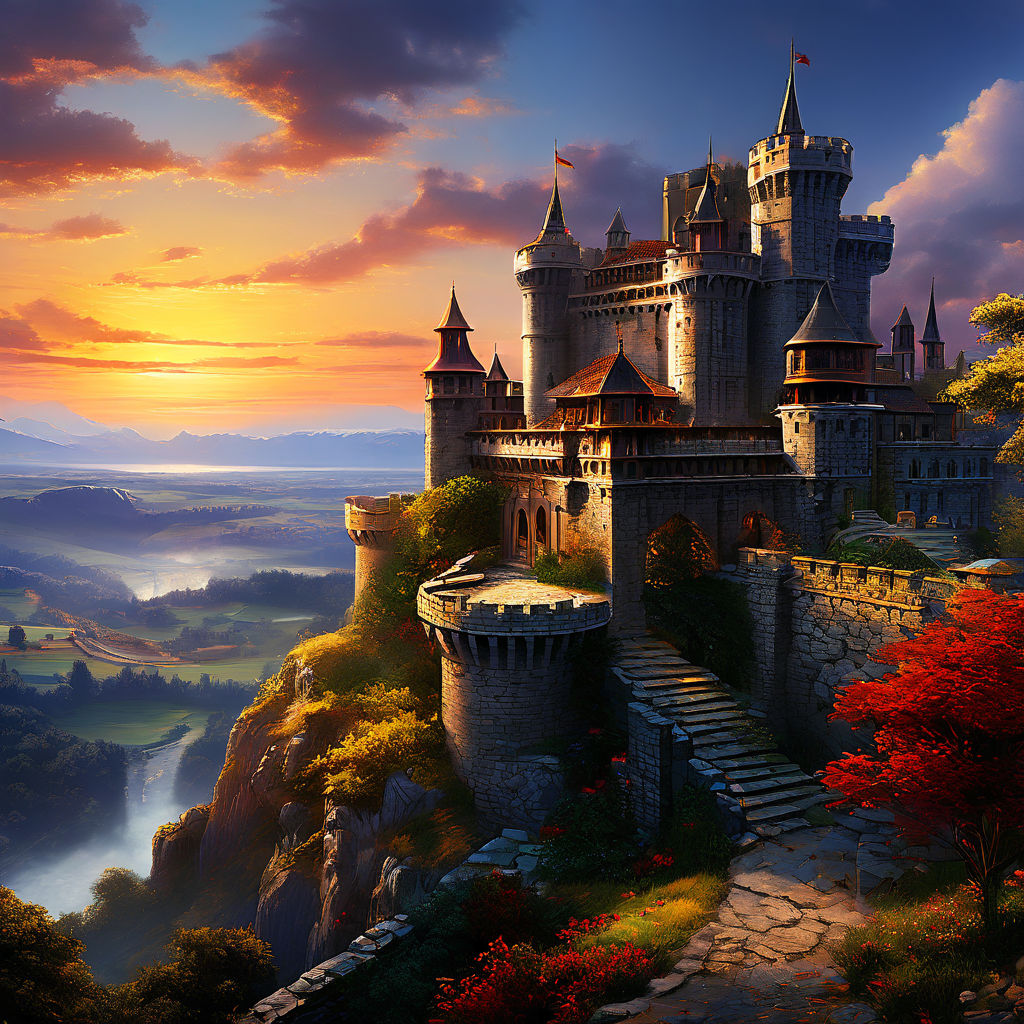The image depicts a stunning, computer-generated castle perched high on a hill during the fall season. The castle, characterized by its four distinct layers of elaborate architecture, is constructed from cobblestone and features multiple peaked roofs and varying levels adorned with flags. Surrounded by foliage in hues of bright red and greenish-brown, the environment suggests autumn with changing leaves on the trees encircling the citadel.

The sky above is painted in a mesmerizing gradient of light to dark blues, accentuated by vibrant ribbons of yellow and orange, detailing a striking sunset. Partly cloudy skies add depth to the composition with wisps of dark orange clouds enhancing the beauty of the scene. The setting sun casts a warm glow over the landscape, progressing toward a reddish horizon.

From the bottom right-hand corner, a rock path winds its way up through red flowers and green grass, leading to a grand staircase comprising about twenty steps. These steps ascend past a balcony and potentially into a courtyard, though no visible doorways lead inside. Various arches on the second-floor hint at window placements, contributing to the castle's complex aesthetic.

In the left section of the image, the valley below the castle extends outward showcasing a picturesque view of river-mingled green fields and distant mountains. A waterway meanders through a lush landscape of more trees and farmlands, painting a serene and idyllic backdrop to this enchanting, digital artwork.